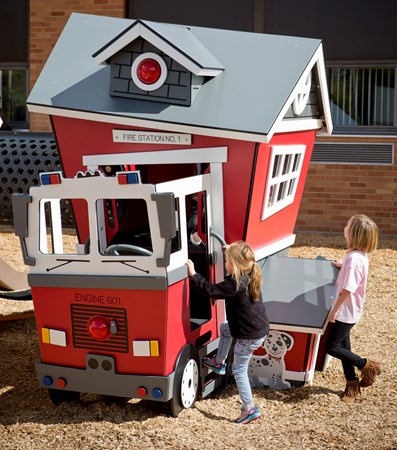In this sunny, real-life photograph of a children's play area, two young girls are depicted playing on a whimsically styled, asymmetrical toy fire station and truck playhouse. The structure is primarily red with a gray roof and sits on a patch of wood chips. The playhouse features a lopsided design giving it a fantastical appearance, with a slanted triangle roof and a front door that tilts downwards on one side. Above the entrance, the sign reads "Fire Station Number 1," and the attached toy fire truck, which is kid-sized and red, displays the text "Engine 601."

One girl, with long blonde hair, is actively climbing into the cab of the truck, while the other girl, with short brown hair, stands looking up at a window of the playhouse. Adding to the charm, a small wood cut-out of a Dalmatian is positioned on the lower part of the fire truck playhouse. The sun's brightness reflects off parts of the play structure, emphasizing the cheerful outdoor setting. There are no other visible people or additional signage in the image.